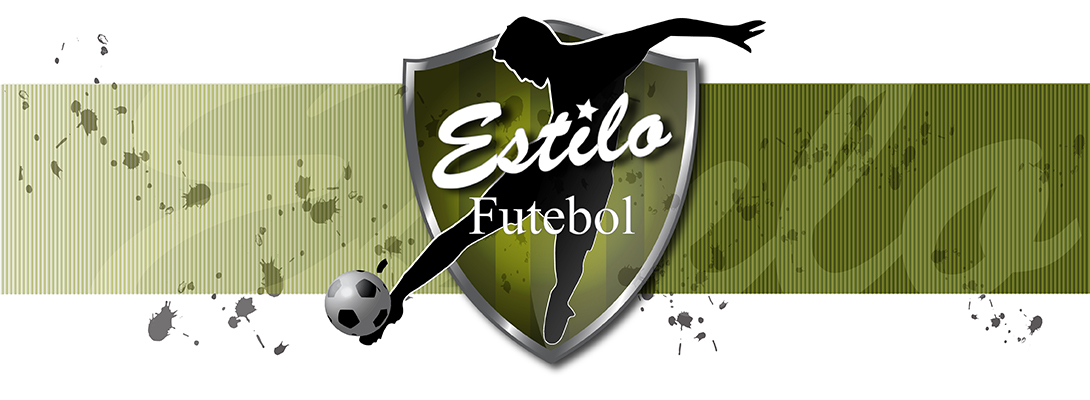A dynamic logo for Estilo Futebol features prominently in the center of the image. The background consists of a green gradient bar that transitions from a light green on the left to a darker green on the right, overlaid with thin vertical lines and textured with splatters of grayish-blue mud. At the center lies a shield crest with alternating vertical stripes of light and dark green and a gray outline. 

Dominating the crest is the black silhouette of a man in the midst of kicking a soccer ball with his right foot. The soccer player is accentuated with a white outline, creating a striking visual against the green background. His left arm is raised to the height of his head, which is tilted down toward the ball making contact with his right foot, while his left foot points straight down toward the pointed end of the shield. 

Overlayed on the man, the word "Estilo" is elegantly written in large white cursive letters, with a five-pointed star dotting the "i". Beneath it, in a bold, non-cursive font, the word "Futebol" is displayed. Overall, the design of the logo captures both the dynamic movement of soccer and the stylistic elements of the brand Estilo Futebol.